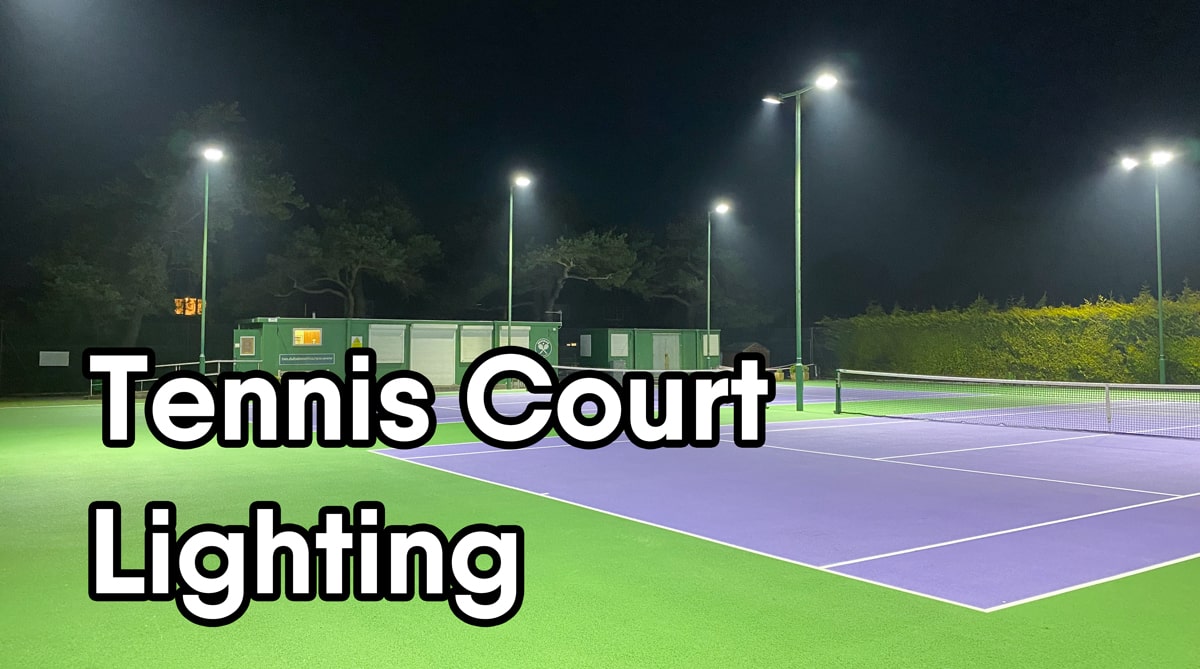This image is an outdoor, nighttime photo of a well-illuminated tennis court. The court itself is painted a distinctive bluish-purple color with crisply marked white lines. Surrounding the court is a lush area featuring green grass, dark green trees, and numerous shrubs. Prominent greenish-yellow poles support bright white lights that effectively illuminate the area, making the scene almost as bright as day. In the foreground, large white letters spell out "Tennis Court Lighting," suggesting the photo is advertising various lighting solutions. Towards the center and back of the image, several green buildings with white doors, windows, and shutters are visible. A few unidentified, rectangular yellow shapes with red writing can also be seen in this area. Enclosing the tennis court is a mix of fences and walls covered in dense foliage, with additional light poles scattered around, particularly noticeable to the right and back. The sky above is pitch black with no visible stars, emphasizing the contrast between the well-lit court and the dark surroundings.